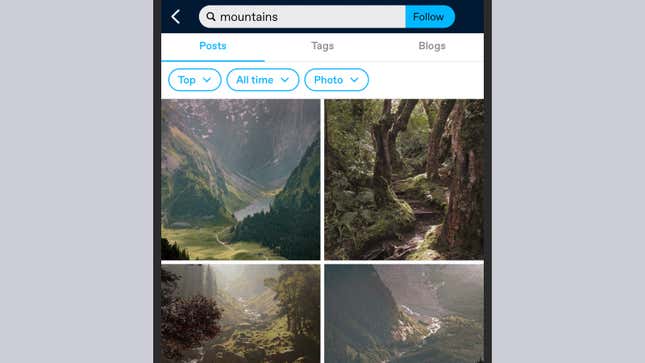The image appears to be a screenshot from a mobile device displaying a search for "mountains" within a blogging or social media application. At the top of the screen, a standard search bar shows the queried term "mountains," next to which there's a "follow" button, suggesting the search is tied to a user or topical category. The predominant background is dark, almost black, creating a strong contrast with the various interface elements.

Directly below the search bar are several filter categories labeled "Posts," "Tags," and "Blogs," written in bright cyan blue text. These categories are followed by additional sorting options: "Top," with a drop-down arrow for further refinement, and "All Time," also featuring a drop-down menu. These sorting options are visibly highlighted in the same bright cyan blue color.

Beneath these filters and options, thumbnail images of mountains are displayed, many of which showcase tropical scenes, indicating the search results. The images are organized in a grid-like format, typical of many image search interfaces. The combination of bright text and vivid mountain imagery against the dark background provides a visually striking interface for users searching for mountain-related content on their mobile devices.